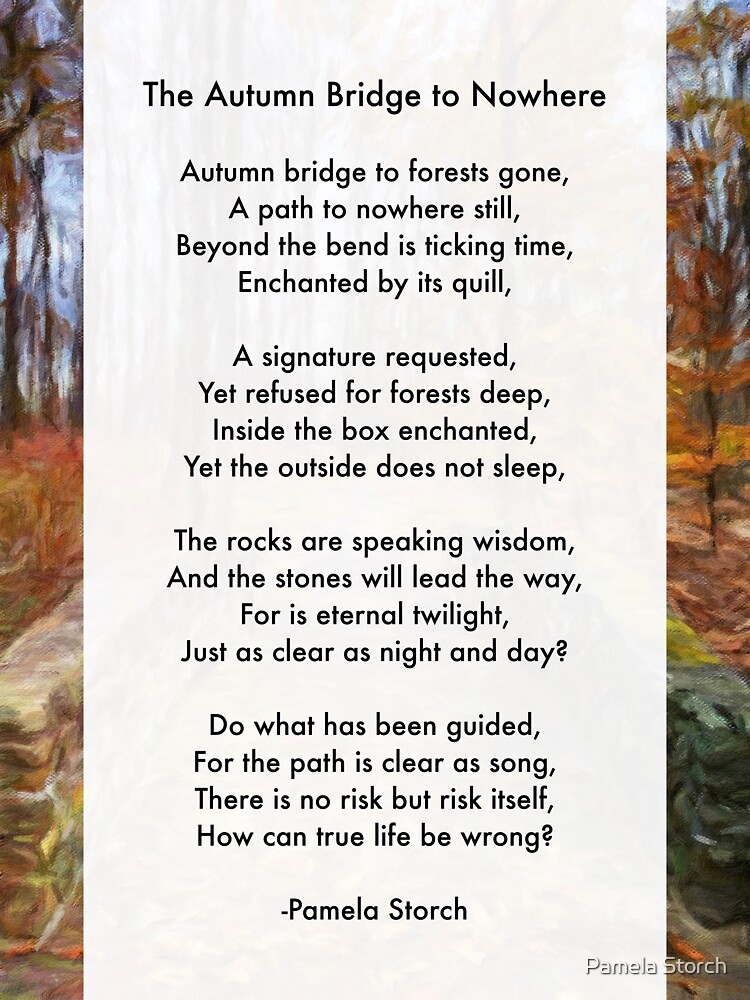The image features a poem titled "The Autumn Bridge to Nowhere" by Pamela Storch, displayed in black letters on a white background. The poem is divided into four stanzas, with the first stanza reading: "Autumn bridge to forest gone, a path to nowhere still, beyond the bend is tickling time enchanted by its quill." Two vertical strips on either side of the image depict parts of a forest, evoking an autumn scenery. On the left side, at the bottom, there is a wall with four distinct shapes at the top. On the bottom right-hand side, you see another wall with the shape of a tree in the background, displaying fall colors. The author's name, Pamela Storch, is written at the bottom in black letters.